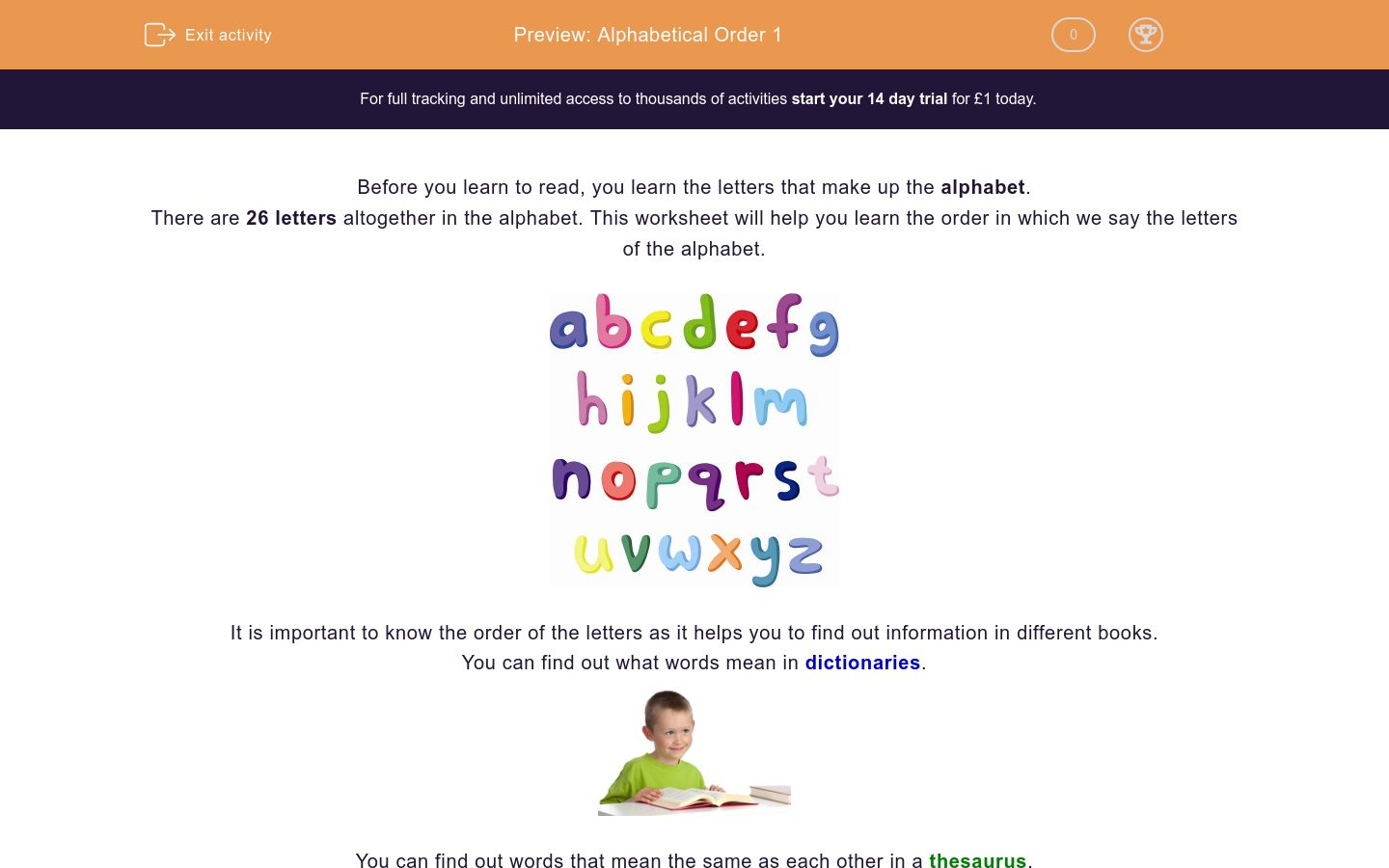The image showcases an educational website interface aimed at teaching the alphabet in alphabetical order. At the top of the interface, there is a header bar with an "exit activity" button. The title "Preview Alphabetical Order 1" is prominently displayed next to a trophy symbol, indicating some level of achievement.

Below the header, there is a dark, greyish-black bar with a message encouraging users to start a 14-day trial for full tracking and unlimited access to thousands of activities, priced at one pound.

The main content area of the webpage is white, and contains a paragraph in small writing that reads: "Before you learn to read, you learn the letters that make up the alphabet. There are 26 letters altogether in the alphabet. This worksheet will help you learn the order in which we save the letters of the alphabet."

Further down, the alphabet is displayed across four rows, with each letter in a different vibrant color. Additionally, there is an engaging image of a small child attentively looking at an open book, reinforcing the educational theme of the activity.